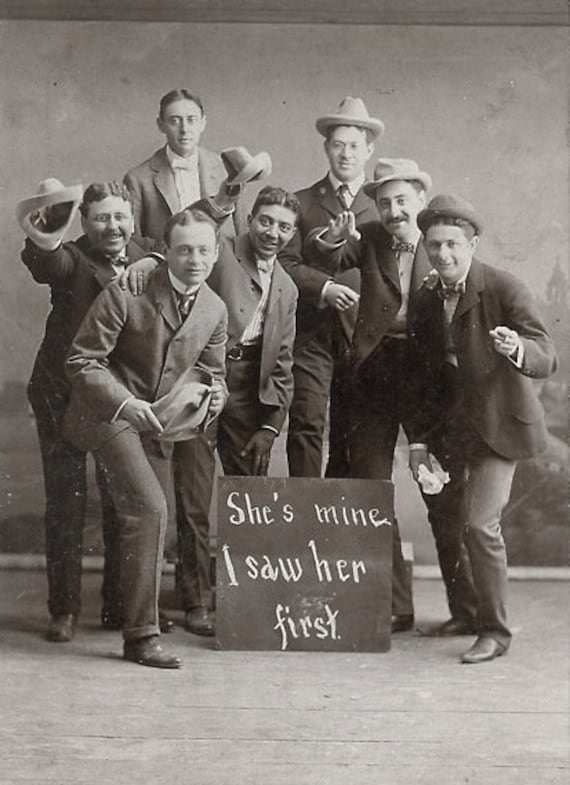In this black and white photograph, there are seven men standing on a wooden slat floor, possibly from the early 20th century or late 19th century. They are all dressed in suits, some with bow ties and others with traditional ties, their jackets either buttoned or unbuttoned accordingly. Several among them wear cowboy-style or straw hats, while others hold their hats in their hands, gesturing towards the camera with exaggerated, broadly smiling expressions, suggesting a jovial or comical mood. The backdrop appears to be a painted canvas, perhaps indicative of a photography studio setting the scene. At their feet is a small square chalkboard with the text "She's mine, I saw her first" written in white chalk, adding a humorous or playful element to the image.